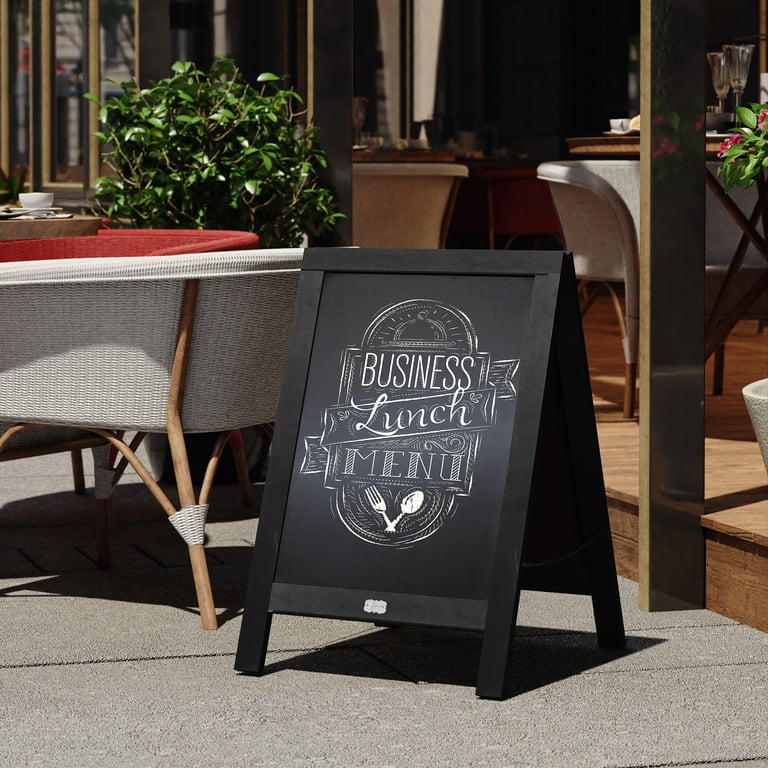This photograph, taken outdoors during the daytime, captures the scene in front of a restaurant. At the center of the image stands a black, foldable billboard sign on a concrete floor. The sign, with professional and modern styling, features white lettering that reads "Business Lunch Menu," accompanied by an intertwined fork and spoon graphic beneath the text, adding a touch of personality.

To the left of the sign, there is a white chair with wicker legs followed by a red chair. Behind these chairs, a small potted bush can be seen. The ground immediately in front is paved with gray stone, leading up to a higher patio area about a foot off the ground. This wooden patio hosts additional chairs and tables, including a beige chair and a table with two wine glasses. Nearby, the corner of another plant with red flowers is visible. As you look further into the restaurant, it transitions to a darker interior, indicating an inviting indoor area beyond the outdoor patio setup. The overall atmosphere suggests a welcoming, versatile dining space suitable for both outdoor and indoor seating.